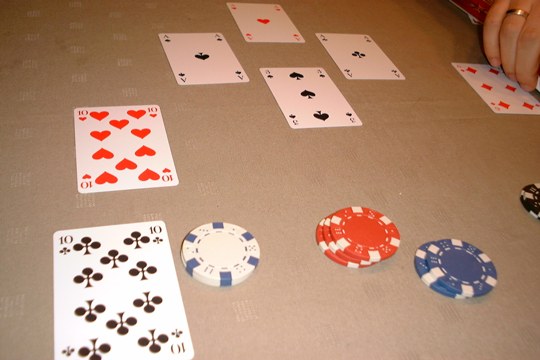This detailed photograph captures the intense atmosphere of a professional poker game. The scene shows a high-stakes competition unfolding on an official poker table, identifiable by its specialized surface and distinct branding. Scattered across the table are multicolored poker chips arranged in neat stacks of orange, blue, black, and white with green edges. 

In the foreground, several cards have been flipped face-up, revealing the six of diamonds, ace of clubs, three of spades, ace of hearts, ace of spades, ten of hearts, and ten of clubs. A player’s hand, adorned with a golden ring, is visible in the upper right corner, poised with a contemplative air over the edge of the table. The angle of the photograph offers a vantage point that could be from the dealer's perspective, showcasing the players seated in a semicircle, deep in the throes of the game. The overall composition and details vividly depict the strategic and calculated nature of professional poker.